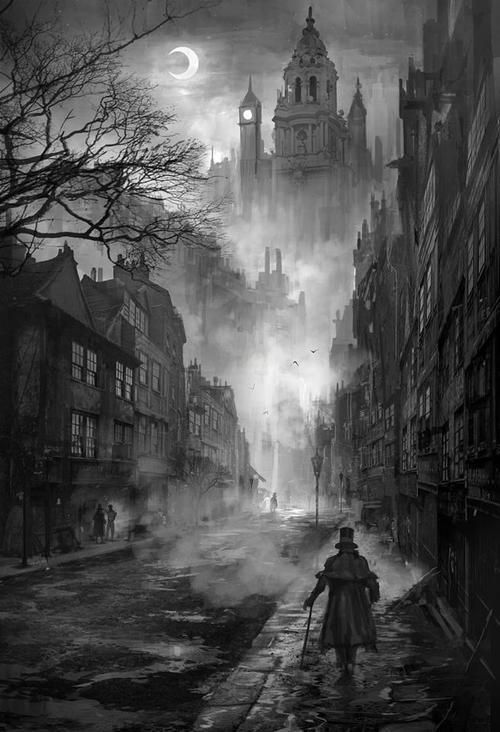The image depicts a detailed, old black and white drawing, imbued with various shades of gray, capturing a foggy nighttime scene in a historic European town. Dominating the forefront on the bottom right, a man cloaked in a dark trench coat and top hat strides along a damp cobblestone walkway, leaning on his cane. Surrounding him, a dense white smog gives an eerie feel to the night, possibly emanating from underground steam or simply the fog descending upon the scene. 

On either side of the street, tall, multiple-story buildings showcase distinct architecture, their shadowy forms partially veiled by the fog. To the left of the man, leafless branches of a barren tree stretch over the street, contributing to the somber atmosphere. Further down the road, two people engage in conversation near an old street light, their figures faintly illuminated in the monochrome gloom.

Ahead, the road ascends towards a colossal, castle-like structure perched on a hill, crowned with a dome and flanked by two prominent towers. The illuminated clock face on one of the towers bears a vague resemblance to Big Ben, peering through the murky fog. High above, a crescent moon hangs in the sky, casting a faint glow over the entire scene while birds glide silently in the distance. Puddles reflecting the dim light hint at the dampness of the street, adding to the mystic, tranquil ambiance of this evocative nocturnal illustration.